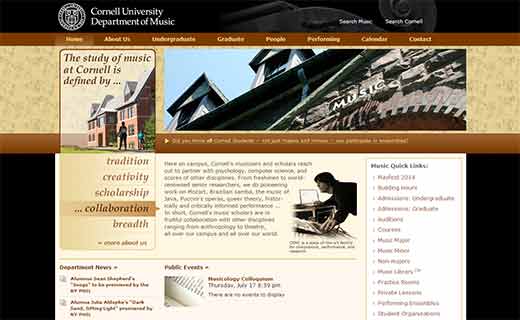Screenshot of the Cornell University Department of Music website. At the top, there's a Cornell University crest followed by the department's name. The navigation menu below includes links for "Home," "About Us," "Undergraduate," "Graduate," "People," "Performing," "Calendar," and "Contact." The introductory text reads, "The study of music at Cornell is defined by..." followed by phrases such as "tradition," "creativity," "scholarship," "collaboration," and "breadth." 

Below this text is an image of a building located on the Cornell campus. Underneath this picture, another phrase is visible: "study of music defined by..." and an image of a person bent over a table, seemingly working on a project. 

On the right-hand side of the page, there is a section labeled "Music Quick Links," which features a list of clickable bullet points. The central part of the page displays a series of brown rectangles at the top and bottom, a beige-colored middle section, and black rectangles on the sides, creating a visually structured layout.